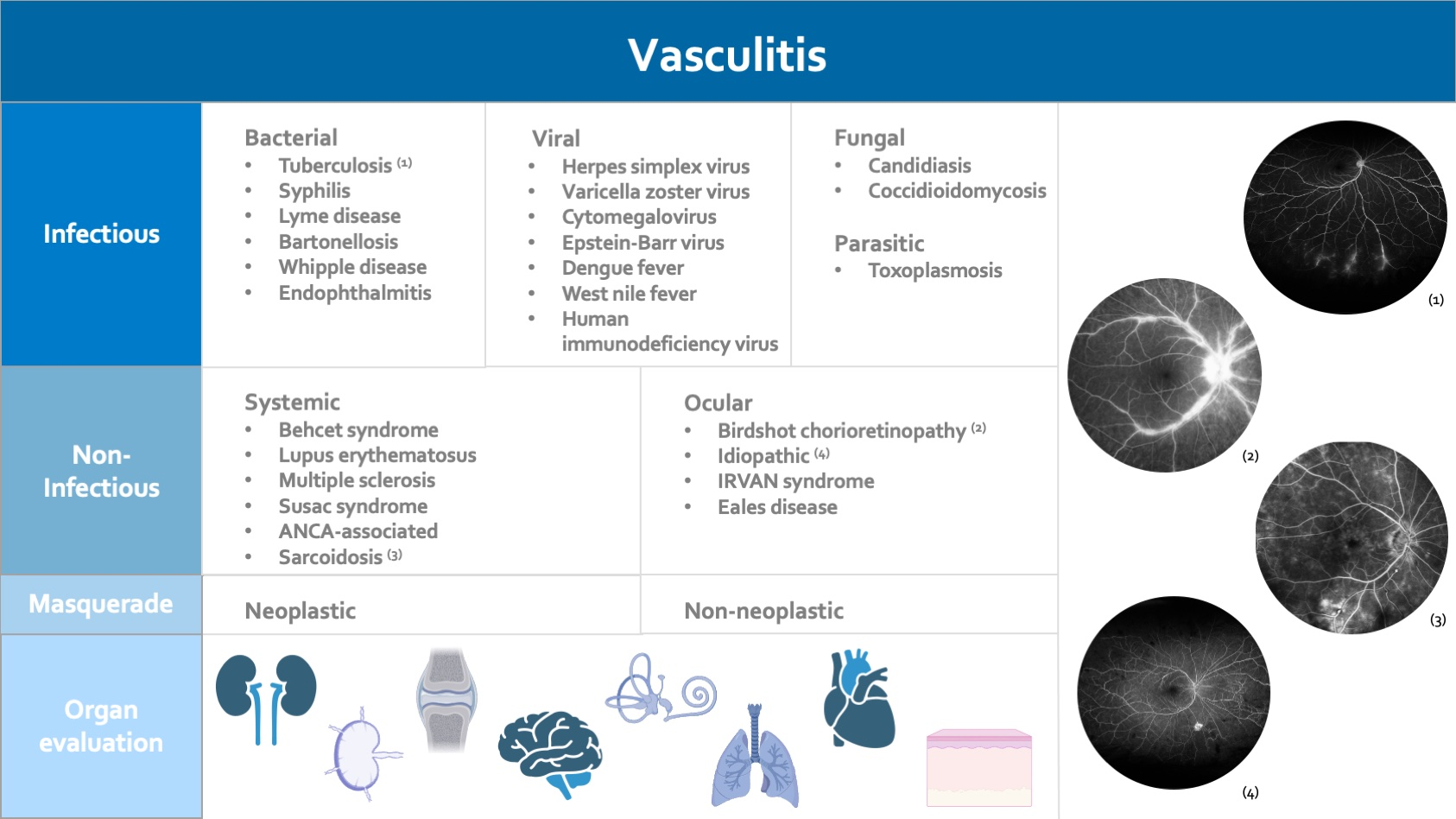The image is an informational poster on vasculitis, predominantly using shades of blue with white and gray text. At the top, it prominently displays the word "Vasculitis" in white on a dark blue background. The poster is segmented into multiple horizontal quadrants, each representing different categories. 

The first quadrant, labeled "Infectious" in a lighter blue, lists three subsections: bacterial, viral, and fungal. Specific diseases mentioned under bacterial include tuberculosis, syphilis, Lyme disease, bartonellosis, Whipple disease, and encephalitis.

Below this, the "Non-Infectious" category is divided into systemic and ocular parts. Systemic conditions included are Behçet's syndrome, lupus, sarcoidosis, and more, although some text here is garbled. The ocular section mentions conditions such as birdshot chorioretinopathy and idiopathic iritis.

The next quadrant, even lighter blue, is titled "Masquerade," subdivided into neoplastic and non-neoplastic categories.

At the lowest section, titled "Organ Evaluation" in the lightest blue, there are icons or thumbnail images of various organs like the heart, lungs, brain, kidneys, and liver, indicating areas potentially affected by vasculitis. Additional black and white circular images of internal organs are placed on the right side, illustrating the condition's impact on these structures.

Overall, the poster provides a comprehensive breakdown of vasculitis, highlighting its infectious and non-infectious causes, conditions that can mimic the disease, and the organs that can be evaluated for symptoms.